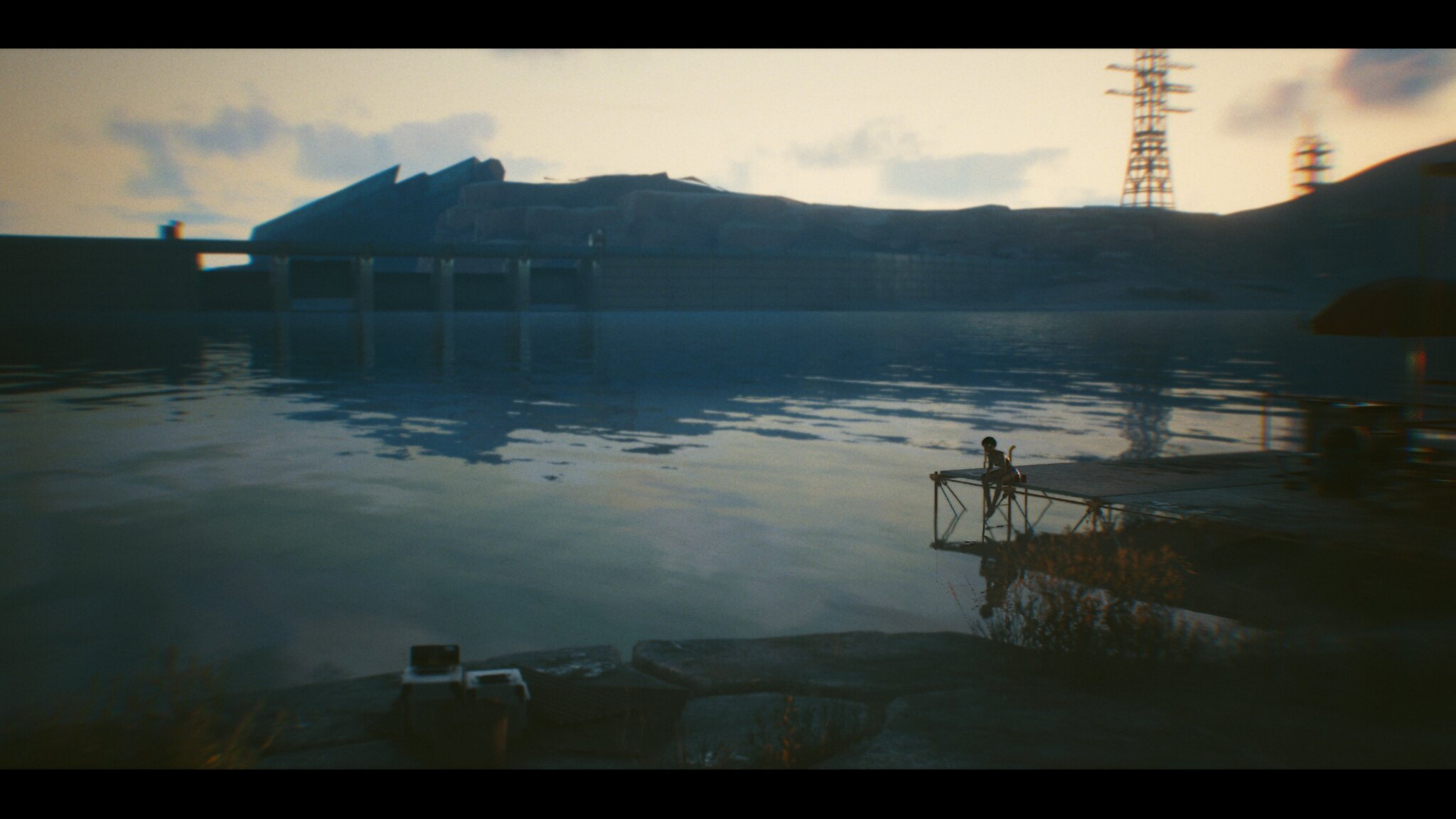A slightly blurred outdoor photograph captures a serene lakeside setting, possibly near a dam. In the middle-right of the image, an umbrella shades a table and several chairs, creating a cozy gathering spot. In the immediate foreground, one or two individuals sit on the side of a flat dock, complementing additional chairs that are positioned to face the tranquil lake. The backdrop reveals imposing elements: in the top right, structures resembling electrical transformer towers or cell phone towers rise against the sky; beneath them, the rock walls and abutments hint at the presence of dam gates. The overall composition blends natural beauty with industrial elements, forming a peaceful yet intriguing scene.